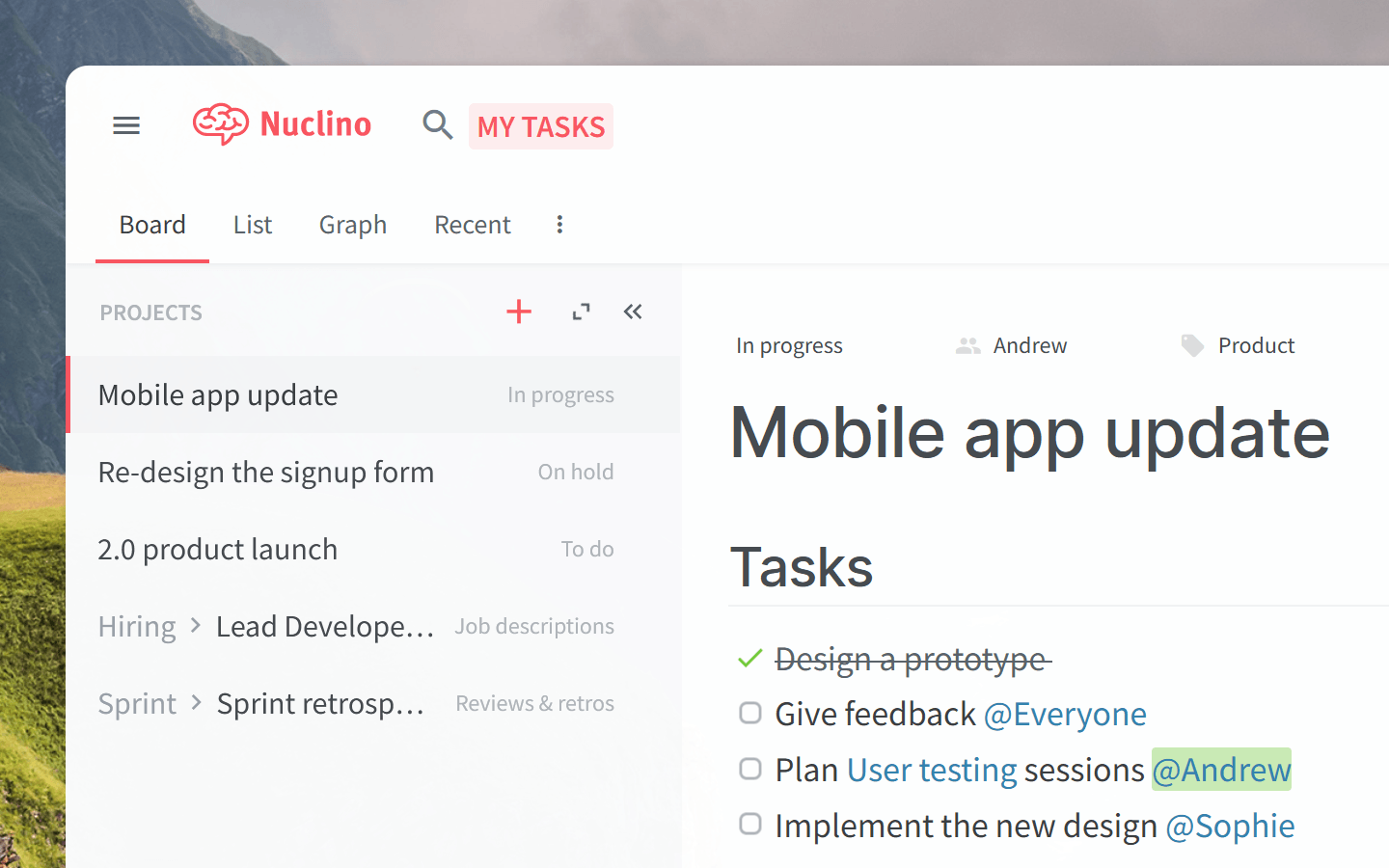In the image, we see the interface of an application identified as "Nucilino" (spelled N-U-C-L-I-N-O), which is indicated in the upper left corner alongside a brain icon symbolizing the app. The background depicts a picturesque scene featuring a green, rolling hill.

The focal point of the image is an open window within the application, specifically displaying the "Mobile App Update" section. Below the "Nucilino" title, there is a vertical navigation menu with various tabs such as "Board," "List," "Graph," and "Recent." Under these tabs, we find the "Projects" section, which highlights that the "Mobile App Update" is currently "In Progress."

In the main window to the right, details related to the "Mobile App Update" project are shown. This section lists four tasks associated with the update, with "Design a Prototype" marked as completed, signified by a checked box.